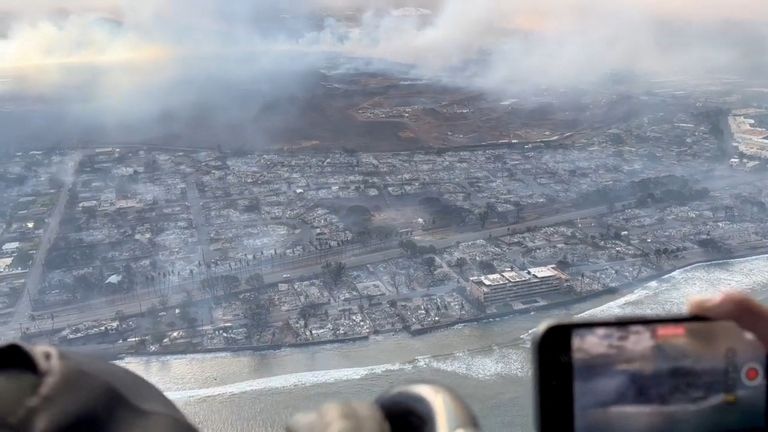The image showcases an aerial view of a small beach town, likely taken from an observatory tower, airplane, or helicopter. The top of the image features a white sky filled with clouds or fog, creating a misty backdrop. Below the sky, a dark grey and brown landscape comes into view, encompassing a small town with primarily grey, concrete buildings. The town is nestled near a shoreline with visible waves crashing onto the beach.

The foreground is dominated by a person holding a smartphone in landscape mode, capturing the scene. The phone screen displays the same view being described, with a blur from the finger covering part of the frame. Several roads traverse the town, with a main highway and smaller residential streets interspersed with an array of buildings and trees. The middle ground shows a bustling cityscape meeting the coastline, with a few white buildings near the water.

Further into the background, the city extends towards a large hill or mountain shrouded in dense mist or smoke. The scene may be during sunrise or sunset, lending a dim light to the overall grey tone of the photograph. Palm trees suggest the location could be in Florida or California. The combination of natural and urban landscapes with visible water below adds richness to this coastal aerial perspective.